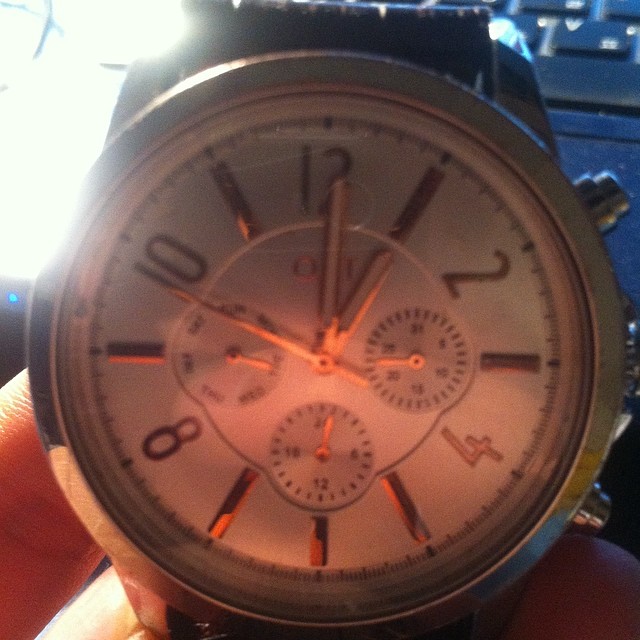The watch features a sophisticated design with a silver rim and a pristine white face, elegantly adorned with gold numbering. The numbers 12, 2, 4, 8, and 10 are prominently displayed, while minimalist lines mark the remaining hours. At the center of the face, multiple smaller dials indicate seconds, directions, and months, providing a comprehensive array of timekeeping functions. The hour and minute hands are long rectangles, gold-edged with white centers, complemented by a gold second hand. A burst of bright light illuminates the upper left corner of the image, likely from an external light source. The fingertips of the person, a Caucasian, holding the watch are visible, along with glimpses of what appears to be a brown leather watch band.